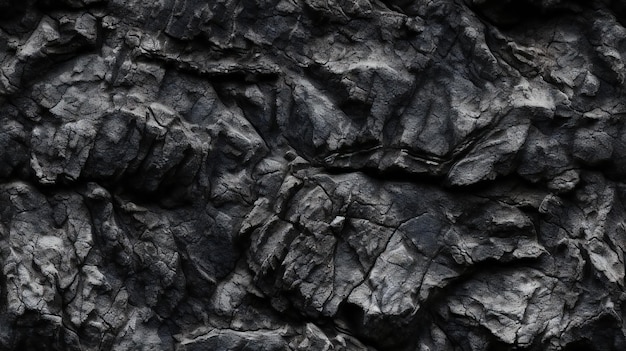The image is a close-up, horizontal rectangular photograph that prominently features a dark, uneven surface, rich in texture and varying shades of black, gray, and white. The subject appears to be a natural formation, possibly a rock face or cliff, characterized by its predominantly smooth, dark gray and black surfaces with numerous ridges, cracks, and bumps resulting from erosion over time. These surface variations create an impression of harshness and sharpness, with certain areas appearing almost sculpted or carved, suggesting possible illusions of faces or animals. The overall appearance is highly textured, akin to charred or heavily burned wood, further contributing to the rugged and jagged visual impact. There is no vegetation, light, or sky visible, focusing solely on the intricate details and natural randomness of this geological feature.